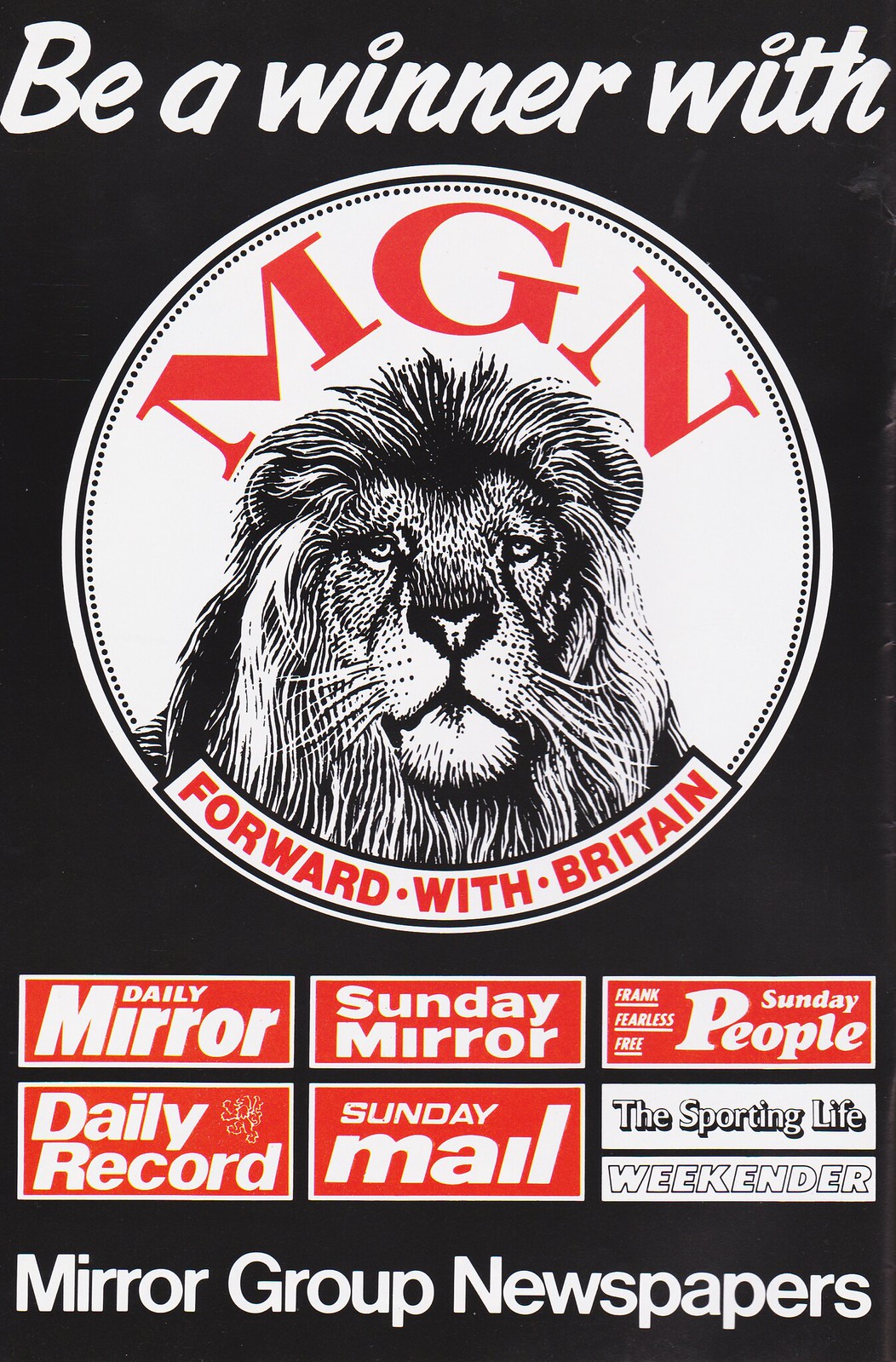The promotional image is an advertisement for the British newspaper conglomerate, Mirror Group Newspapers (MGN). It features a sleek black background with prominent white and red text. At the top, in italicized white letters, the ad encourages readers to "Be a Winner With." Below this slogan is a large, eye-catching white circle encased in a black ring, prominently featuring a meticulously hand-drawn black-and-white sketch of a lion's face, looking straight ahead.

Above the lion, in bold red letters, it reads "M-G-N," and directly beneath the lion's powerful gaze, the slogan "Forward with Britain" is displayed in red text. Further down the ad, there is a three-column by two-row grid layout containing red boxes with white text, except for the last box which is in black and white. These boxes list the newspapers under the Mirror Group. From left to right, the first row includes "Daily Mirror," "Sunday Mirror," and "Sunday People" alongside the phrase "Frank Fearless Free." The second row lists "Daily Record," "Sunday Mail," and "The Sporting Life Weekender." 

At the very bottom of the advert, in crisp white letters, the ad concludes with "Mirror Group Newspapers," succinctly summarizing the conglomerate's brand presence.